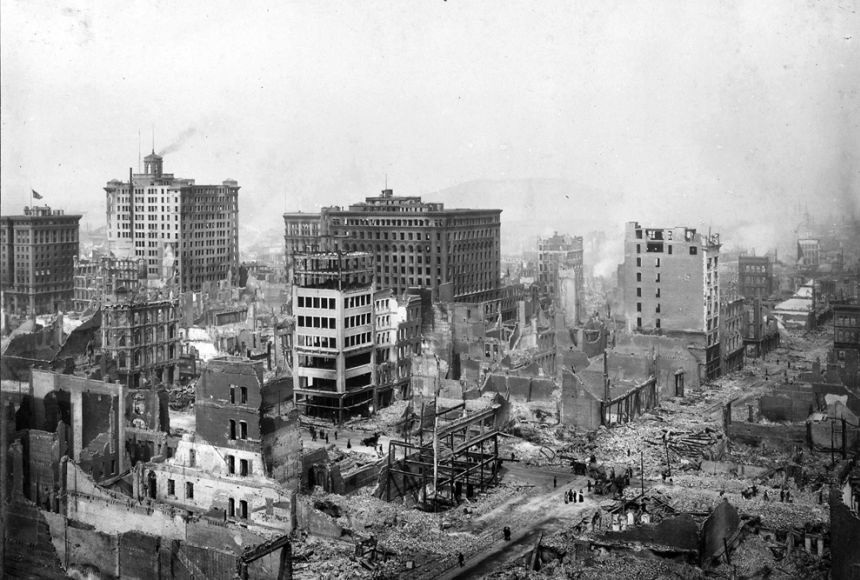The black and white photo, likely from the early 1900s, captures an elevated, overhead view of a city in disarray. The landscape layout is predominantly filled with crumbling buildings and debris-strewn streets, suggesting the aftermath of a disastrous event, possibly a fire or bombings. The top half of the image shows a hazy, white expanse which could be smoke rather than sky, hinting at the recent devastation. In the foreground, one particularly dilapidated building stands out amongst the various tall structures. Amidst the ruins, some trees and scattered dark spots, which could be ash, are visible, adding to the stark ambiance of the scene. The overall impression is one of an old, ravaged city, frozen in a moment of chaos and destruction.